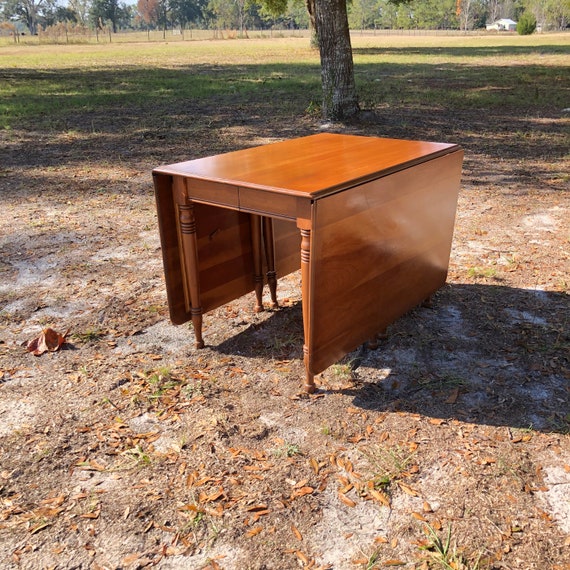In the image, a wooden, brown, and exceptionally clean dining table with dropped sides stands in the middle of a bare field. The main section of the field is devoid of grass, while the background gradually transitions to a grassy area. A solitary tree, appearing somewhat lifeless, is seen prominently in the foreground, providing a stark contrast to the more vibrant trees scattered in the distance. To the right side of the image, a small residential house is visible, partially obscured by bushes, and there appears to be a wire or metal fence marking the boundary of the yard. The table, reminiscent of those found in hotels with extendable flaps, is placed peculiarly in this outdoor setting, adding an element of surreal juxtaposition to the serene, slightly chaotic landscape marked by fallen leaves.